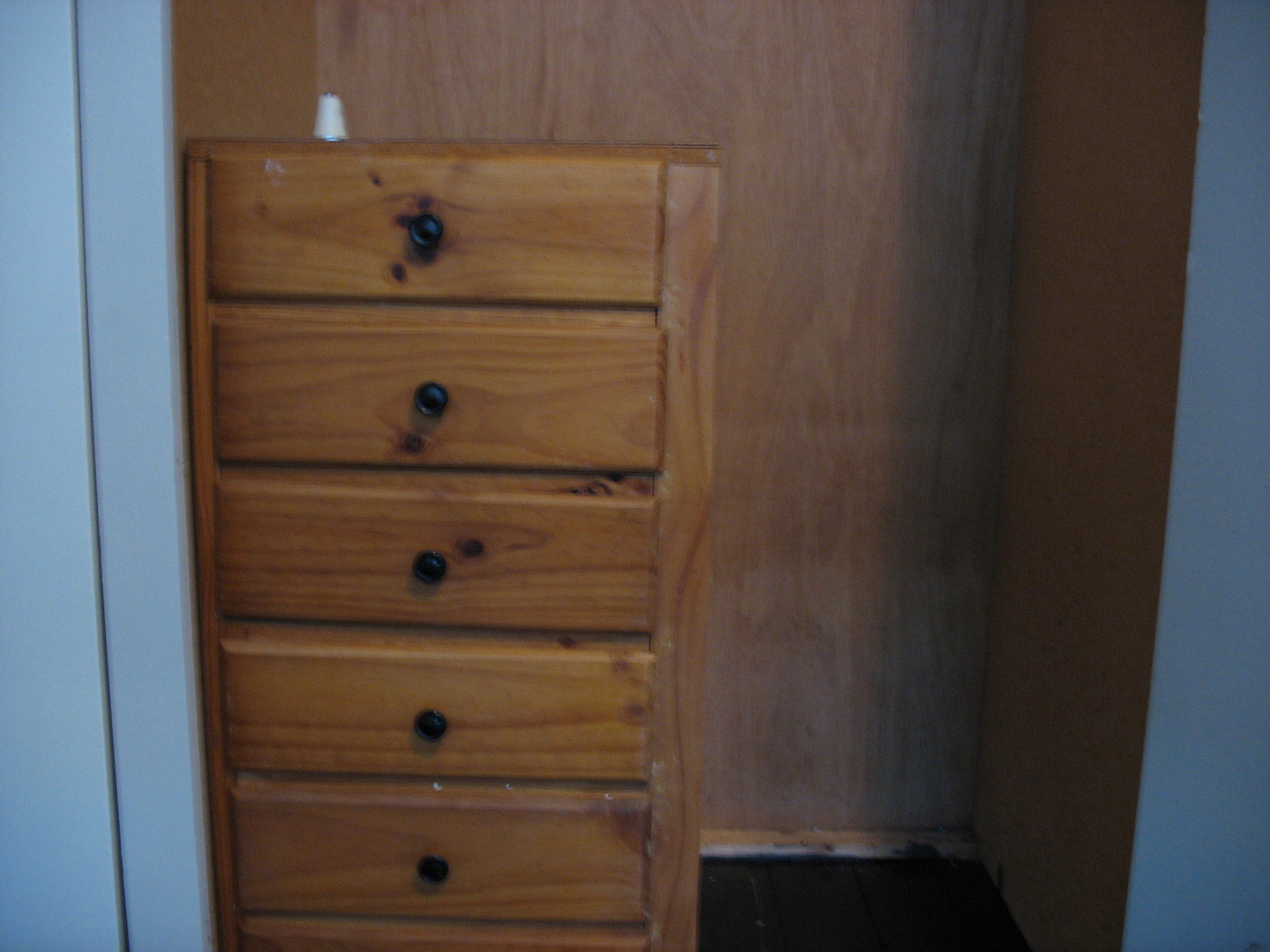In this indoor image, we see a recessed nook or closet space with no doors, situated in a room with blue walls. The back and side walls of this nook are made of lighter, slightly tanned wood, potentially plywood, and the floor is a rich, dark brown. Inside this nook sits a prominent wooden dresser with a grainy oak finish and five drawers, each adorned with a single black brass handle. The chest is positioned a bit crookedly within the space. On the top left corner of the dresser rests a white device, likely an air freshener, designed to keep the room smelling pleasant. There's a small white stain on the top drawer’s left corner. Observably, there are no baseboards on the floor, adding to the slightly unfinished look of the area. Surrounding the recessed nook, the room features white walls with visible trim in the bottom left-hand corner, suggestive of a door frame. The main emphasis of the photograph is this well-crafted, solid wood dresser tucked into the otherwise empty nook, creating a simple yet functional setup.